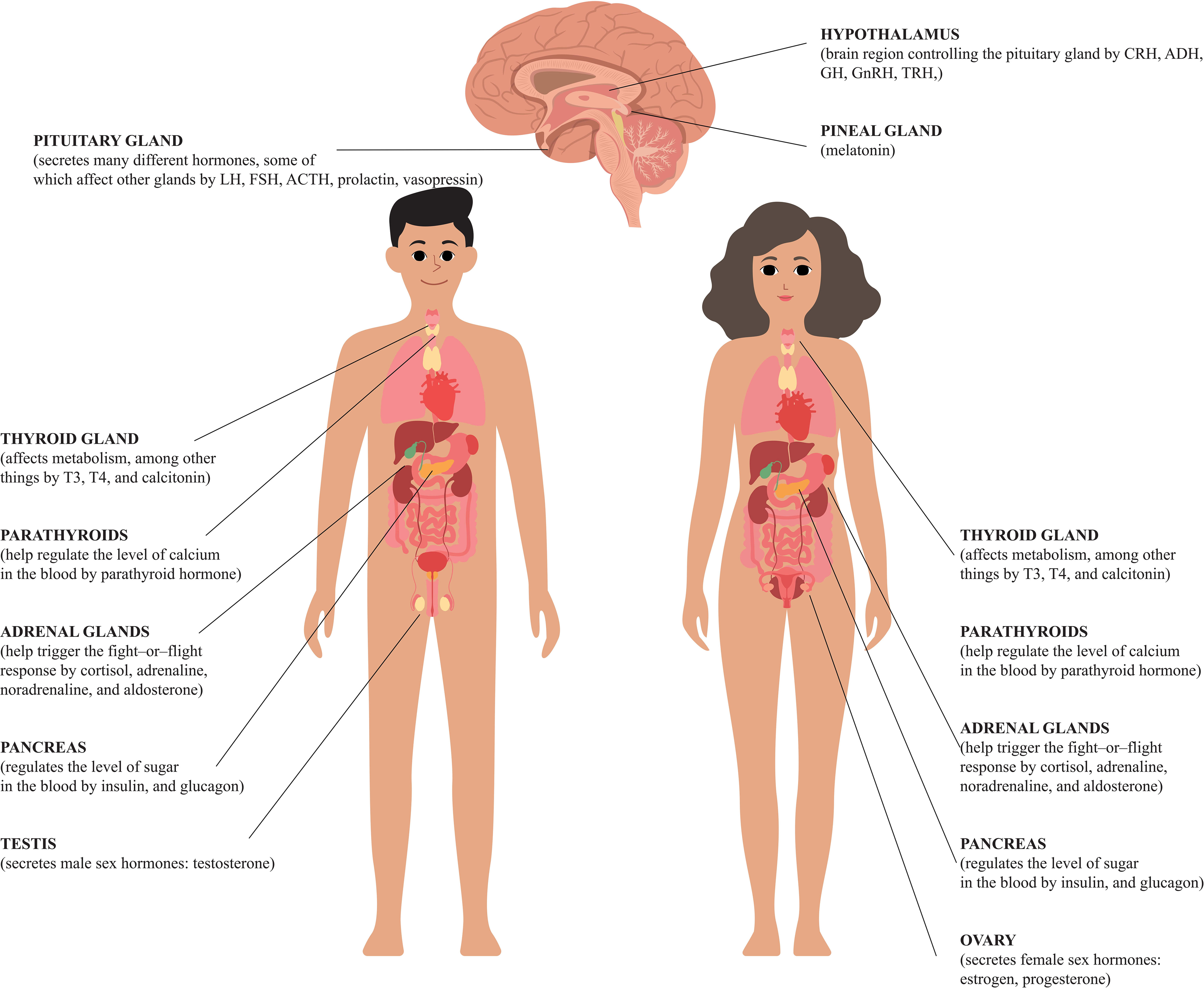The image is a detailed, stylized color diagram illustrating the endocrine systems of a man and a woman. At the top, there's a drawing of a brain highlighting the hypothalamus, pineal gland, and pituitary gland. Below the brain, the diagram splits into two sections: the left side features a man and the right side a woman, both depicted in light beige with their internal organs shown in different shades of red and brown.

Each figure has specific endocrine glands labeled: the thyroid, parathyroids, adrenal glands, and pancreas. Additionally, the male figure has the testes labeled, while the female figure highlights the ovaries. These glands are outlined transparently within the cartoon-like bodies to indicate their locations clearly. The diagram includes brief descriptions explaining the function of each gland, tailored specifically to their role in either the male or female body.